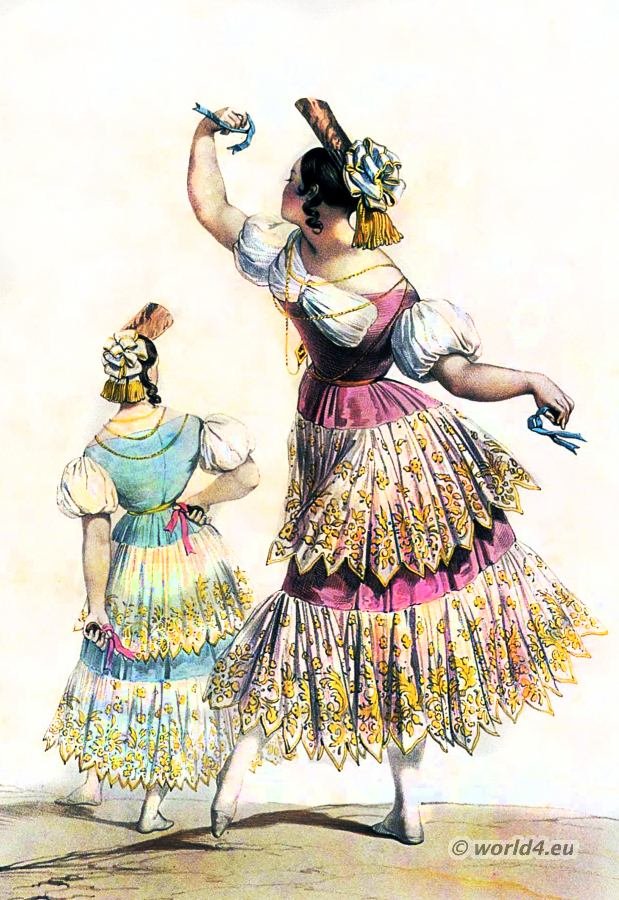The illustration features two Spanish women dressed in traditional 1836 Bolero dance costumes, engaging in a graceful dance. The setting is indicative of traditional choreography with a vintage fashion illustration style, rendered in color and in portrait orientation. The background is a creamy white, while the ground appears beige or brownish in color.

The central figure, the larger of the two women, wears an elaborate pink and white dress adorned with floral frills and two ruffled tiers. Her bodice is a dark rose color, with white puffy off-shoulder sleeves, and she accessorizes with a rolled brown fabric and a bow atop her black hair. This dancer has her right hand elegantly raised above her head, holding a small gray flower, while her left hand gently holds the fabric of her dress. One of her feet is firmly planted on the ground, while the other is poised with pointed toes, capturing her mid-dance. 

To her left stands another woman, smaller in stature, attired in a similar blue and white outfit. She too wears a traditional headdress with short hair curled on the sides, facing away from the viewer in a dance stance with her back to us. At the bottom right of the image is a hashtag and copyright marking that reads "world4.eu" in brown text, completing the vintage and detailed aesthetic of this traditional Spanish dance scene.